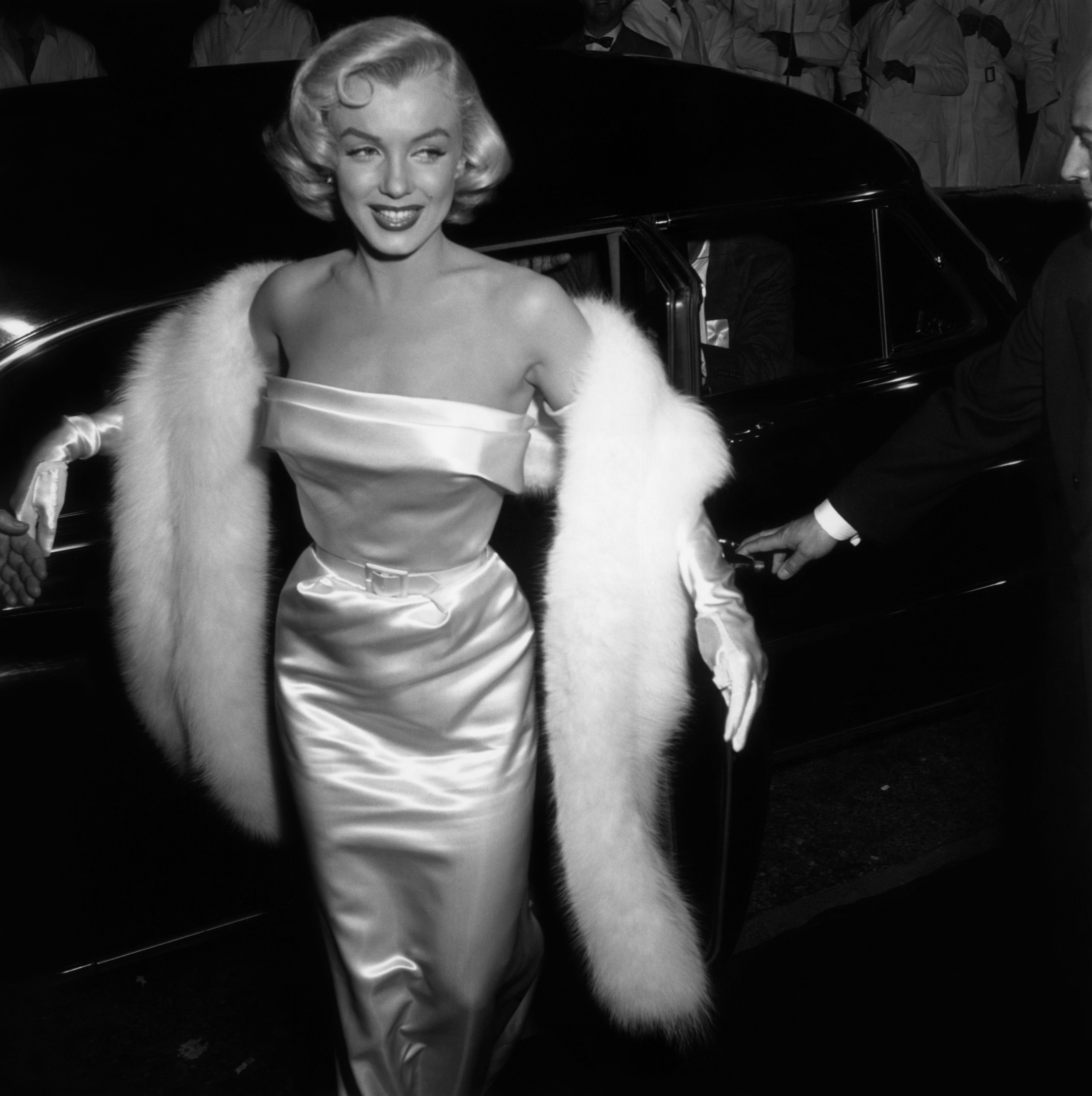This vintage black-and-white photograph, vertically rectangular in format, captures Marilyn Monroe outdoors at night, illuminated by artificial light. Marilyn, adorned in a white satin, ankle-length strapless dress that features a cuff at the top and a matching belt at the waist, is facing the viewer with a gentle smile, her blonde curls styled around her face and forehead. She is embellished with heavy makeup and accessorized with long elbow-length satin gloves. Draped over her shoulders, hanging down both sides of her body, is a luxurious white fur stole. To her right, a black sedan serves as a part of the backdrop, with a man partially visible—just the forehead, eyes, nose, and arm—opening or closing the car door for her. Marilyn's left hand appears to be reaching forward, perhaps to take the hand of someone unseen, while her right hand rests on the door behind her. The scene looks poised as if she is either exiting or about to enter the vehicle, adding to the glamorous and candid nature of the moment amidst a dark, indistinct background.